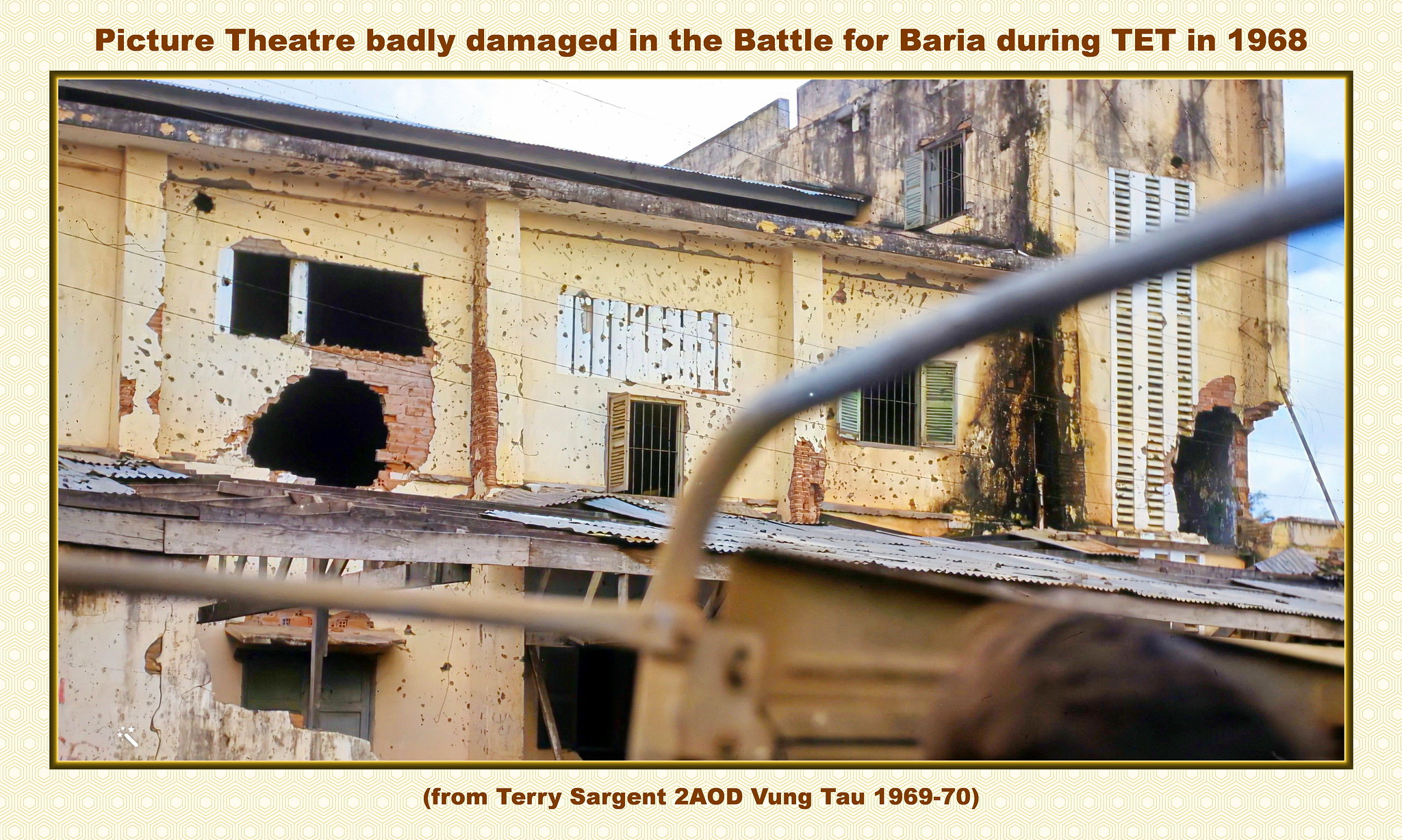The image is a war-torn photograph, almost resembling a poster, with notable text both at the top and bottom. The top of the image reads, "Picture theater badly damaged in the battle for Baria during TET in 1968," while the bottom states, "From Terry Sergeant to A.O.D. Vung Tau 1969-70." The centerpiece of the image is a severely damaged building, primarily showcasing the second floor. The building has a yellow facade marred by significant damage: a large hole under a broken window on the left, and extensive burn marks on the right. The windows are shattered, some boarded up, and bars are seen on the remaining intact window with open yellow shutters. The wall paint is peeling off, revealing patches of brown specks. In front of the main structure, the roof is tin-covered, and the building's lower end is in visible disrepair, with broken wood and numerous holes. Behind this structure stands a taller, even more deteriorated building with significant chunks missing and featuring white vent-like slits. An air conditioner juts out incongruously from one of the boarded windows. The foreground shows a metal bar running diagonally across the image, and part of a person's head is visible at the bottom right. Overall, the photo vividly captures the aftermath of intense conflict and devastation.